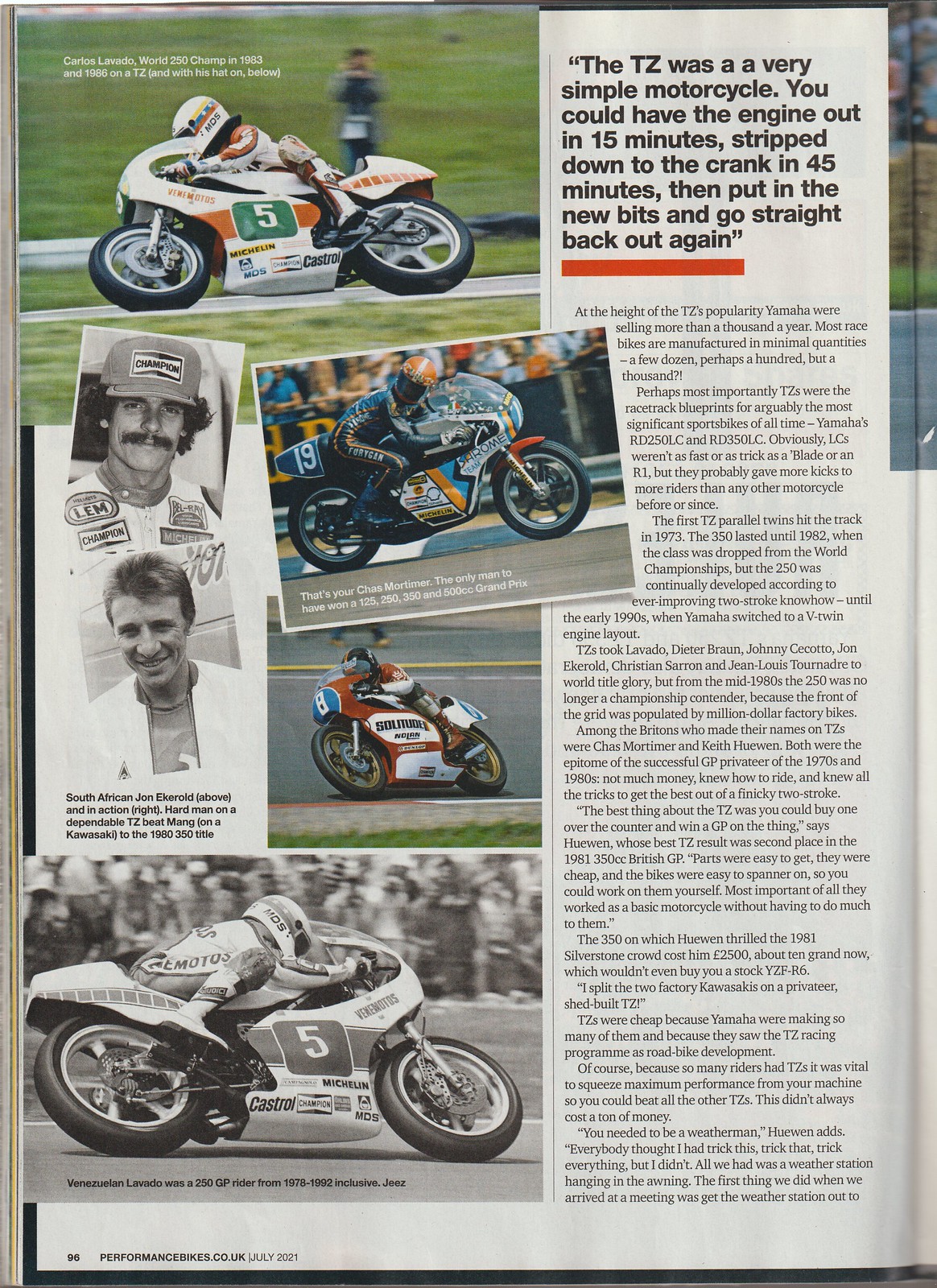The image shows an old vintage page from a magazine focusing on motorcycle racing. On the left-hand side, there are several colored and black-and-white images of motorcycles and their riders. These include close-ups of two men: one with curly black hair wearing a "Champion" cap, and the other, South African John Eckerold, with short light hair in a white jacket. Notable motorcycles depicted include a white motorcycle with orange parts, number five on its front, ridden by Carlos Levedo, a world 250 champion in 1983 and 1986. The text at the bottom mentions that Levedo was a 250 GP rider from 1978 to 1992. Smaller frames show these men leaning nearly flat on their motorcycles as they navigate the racing track. The right-hand side features an article titled "The TZ was a very simple motorcycle," explaining the motorcycle’s easy maintenance: the engine could be removed in 15 minutes and stripped to the crank in 45 minutes for quick repairs. The article continues with further details on the motorcycle's capabilities and racing success.